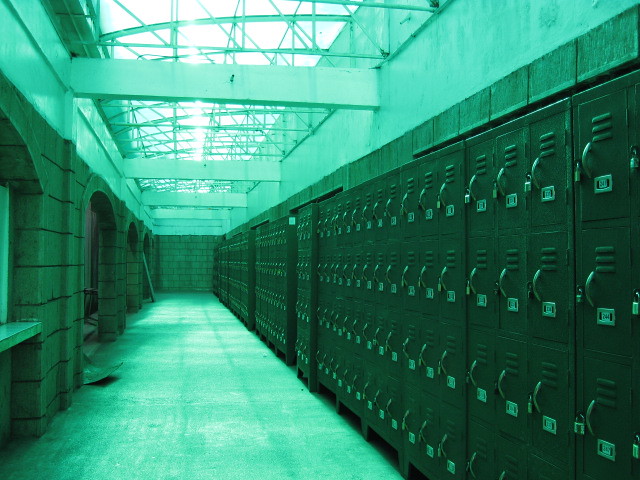This photograph captures the interior of what appears to be a 19th-century train station, bathed in a pervasive green tint that lends the room a somewhat melancholic ambiance. The station features a classic metal-framed skylight, through which sunlight streams, illuminating the space below. On the left side of the image, the structure is characterized by a wall built from stone, complete with large arch entranceways typical of old train stations. The back wall continues the theme with a brick construction. To the right, an extensive row of metal lockers dominates the hallway. Each locker is equipped with a handle, a padlock, a vent, and a number plate, numbering potentially up to 100-200 in total. The ceiling of the hallway reveals a metal grid-like framework, which supports the skylight. This unique combination of architectural elements and the green tint creates a distinctive and somewhat somber visual effect.